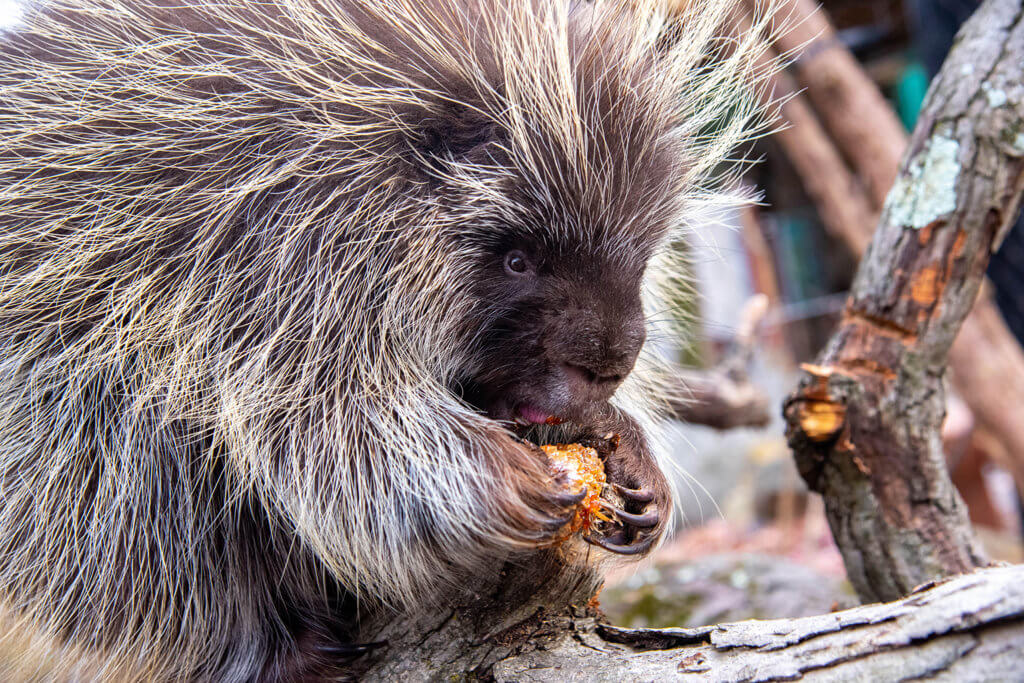The image features a porcupine with a distinctive black face contrasted by an array of white quills that surround its striking eye, which serves as a focal point. The porcupine is holding an orange object, likely a nut or some type of fruit, firmly with its long claws, appearing to be in the process of eating it. The scene includes various pieces of wood and tree bark on the ground, along with another tree angled behind the porcupine. In the background, there's a structure with windows that reflect a blue shine. The setting is detailed with the dry fur and visible back and front claws of the porcupine, emphasizing its natural environment and behavior.